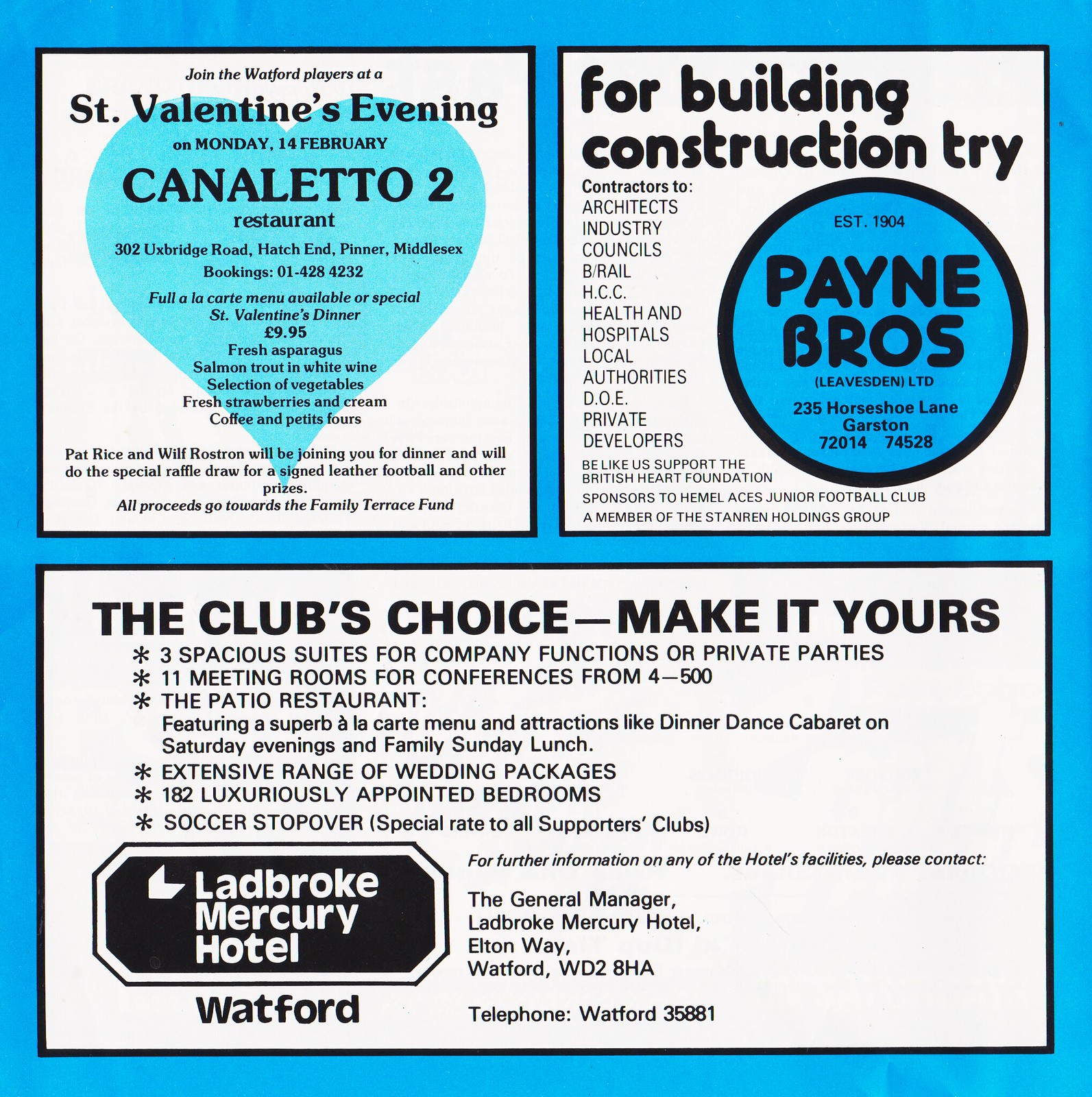This image features a series of three advertisements set against a blue background. The top left ad promotes a St. Valentine's evening event with the Watford players on Monday, February 14th, at Canaletto 2 Restaurant located at 302 Uxbridge Road, Hatch and Pinner Middlesex. The special evening, costing £9.95, offers a full à la carte menu including fresh asparagus, salmon, trout, white wine, a selection of vegetables, fresh strawberries and cream, coffee, and petite fours. Pat Rice and Will Rothschild will be in attendance, participating in a special raffle draw for a signed leather football and other prizes, with all proceeds supporting the Family Terrace Fund.

The top right ad is for Payne Brothers, a building construction company categorized as contractors for architects, industry, councils, the health sector, local authorities, and private developers. The ad highlights their support for the British Heart Foundation and their sponsorship of the Hamill Aces Junior Football Club. It lists their address as 235 Horseshoe Lane, Garson, with contact numbers 72014 and 74528.

The bottom ad features the Ladbroke Mercury Hotel in Watford, promoting its extensive amenities. Highlighted offerings include three spacious suites available for company functions or private parties, 11 meeting rooms suitable for conferences of 4 to 500 people, and the Patio Restaurant which offers superb à la carte menus, dinner dances, cabaret on Saturday evenings, and family Sunday lunches. The hotel also provides an extensive range of wedding packages and 182 luxuriously appointed bedrooms. Additionally, there are special rates for soccer supporters clubs. Contact information is provided for further details on the hotel's facilities, with the address listed as Elton Way, Watford WD2-8HA, and the phone number as Watford 35881.